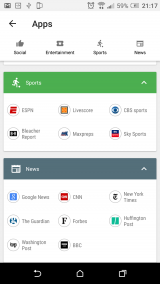### Detailed Caption for the Image

An upright, vertically-oriented yet very blurry screenshot, likely taken from an Android or iPhone device. The frame consists of various navigational and informational elements, making it somewhat difficult to discern.

#### Top Bar:
- **Gray Bar:** This bar sits at the very top, displaying several icons in black.
  - **Icons:** 
    - The first two are indistinguishable squares and rectangles.
    - The third icon is unknown.
    - The fourth icon is an alarm clock.
    - Next to these, there is an icon resembling a circle with lines underneath, its purpose unclear.
- **Wi-Fi Signal Icon:** Indicates connectivity with two out of four bars filled.
- **Battery Indicator:** Shows 59% charge with a partially filled battery icon.
- **Time:** 21:17 is displayed in the upper right corner.

#### Main Screen Content:
- **White Area:** Directly below the gray bar, a large white section dominates the screen.
  - **Rightward-Pointing Black Arrow:** Located on the right side.
  - **Text "Apps":** Displayed in large black letters to the right of the arrow.
- **Icons and Labels:** Below the "Apps" text, several icons and words, albeit blurry:
  - **Thumbs-Up Icon:** Likely labeled "Social" beneath it.
  - **Square Icon:** Filled in white, presumably labeled "Entertainment."
  - **Person Kicking Ball Icon:** Probably labeled "Sports."
  - **Newspaper Icon:** Close to it, with the label "News."

#### Middle Section:
- **Gray Background:** Extending below the initial icons, the middle section is punctuated with a green rectangle featuring:
  - **Sports Emblem:** A figure kicking a ball in white.
  - **Text "Sports":** Displayed in white letters.
  - **Minimize Button:** Indicated by an upward-facing white "V" on the upper right.
- **White Box with Small Icons:**
  - **Top Row:**
    - **ESPN Logo:** Marked with "ESPN."
    - **Orange Square in a Blue Circle Icon:** Likely labeled "Live Score."
    - **CBS Logo:** Followed by "CBS Sports."
  - **Bottom Row:**
    - **Gray-Outlined Circle with Black Box Icon:** Its label is unreadable.
    - **Blue Logo:** Unclear but appears to say "Press."
    - **Blue-Red Circular Icon:** With white text, possibly labeled "Sky Sports."

#### Lower Section:
- **Gray Divider:** Separates the middle section from the next part.
- **Off-Blue Box:** Contains a news icon in white alongside the text "News."
  - **Right Arrow:** An upward-facing white "V."
- **Icons in White Box:**
  - **Top Row:**
    - **Blue Square with 'G':** Marked "Google News."
    - **Red Square Icon:** Presumably "CNN."
    - **Calligraphy 'T':** Labeled "New York Times."
  - **Bottom Row:**
    - **Top Left Icon in Blue Circle:** Likely "The Guardian."
    - **Capital 'F':** Marked "Forbes."
    - **Aqua Blue 'H':** Labeled "Huffington Post."
    - **Washington Post Icon:** Marked by "WP."
    - **Black Square Icon:** Unclear, but probably "BBC."

#### Bottom Bar:
- **Black Bar:** Runs along the very bottom with three key icons.
  - **Left Arrow:** A white curved arrow, possibly a refresh or back button.
  - **Cylinder Outline:** A white icon filled in with black, function unknown.
  - **Square Icon:** White-rimmed and black-filled, likely signaling an app-related function.

Overall, the content layout and icons suggest that this might be a screenshot from an app-related section or a multitasking menu on a smartphone.